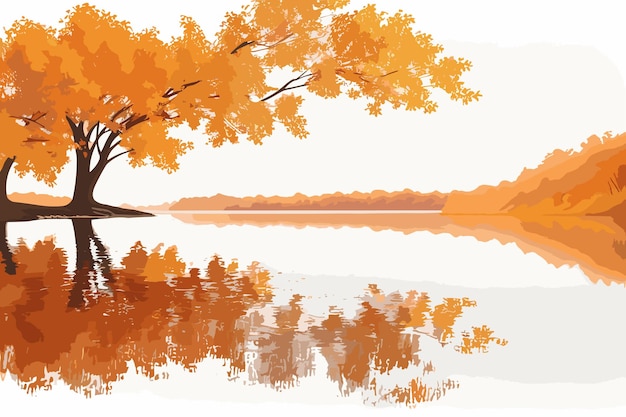This stunning digital artwork depicts a serene, surreal scene dominated by hues of orange and cream. On the left side of the image, a large tree with a long brown trunk and vibrant orange leaves extends its branches across the middle and upper parts of the painting. The tree stands on the bank of a white, reflective body of water, possibly a lake, where the orange leaves and brown trunk create a mirrored image on the water's surface. The backdrop features distant hills or small mountains that continue the theme of orange and are similarly reflected in the still waters. Both the sky and water share a muted white or cream color, adding to the abstract and calm atmosphere. The painting is void of any animals or people, focusing entirely on the enchanting and peaceful autumnal landscape.